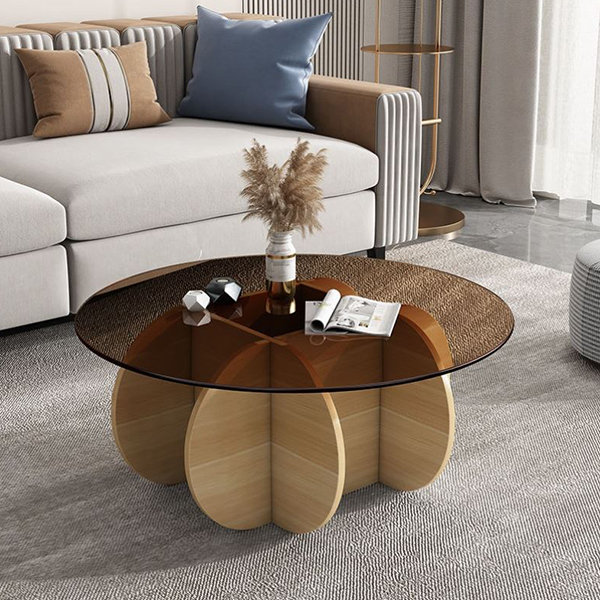This indoor color photograph captures a contemporary living room, with the focal point being a round coffee table at the center of the image. The table has a smoked glass top, tinted brown, resting on a unique, unfinished wooden base composed of four interlocking, pill-shaped slabs that form an intricate, puzzle-like design. On the table, there's an open magazine, a vase with dried, meadow-like flowers, and two faceted candle holders—one slate-colored and one silver. The table sits on a large, short gray area rug.

In the background, a light gray sofa with tufted back and side armrests stretches from the left to the right of the image. The sofa is adorned with a blue cushion and a tan cushion. To the right, in the upper corner of the image, a window covered with sheer curtains filters light into the room. Adjacent to the sofa, a sleek, brass-colored bookshelf with round shelves stands out, and a pouf or footstool peeks into the frame from the right. The floor beneath the rug appears to be a polished, gray stone, completing the modern aesthetic of the space.